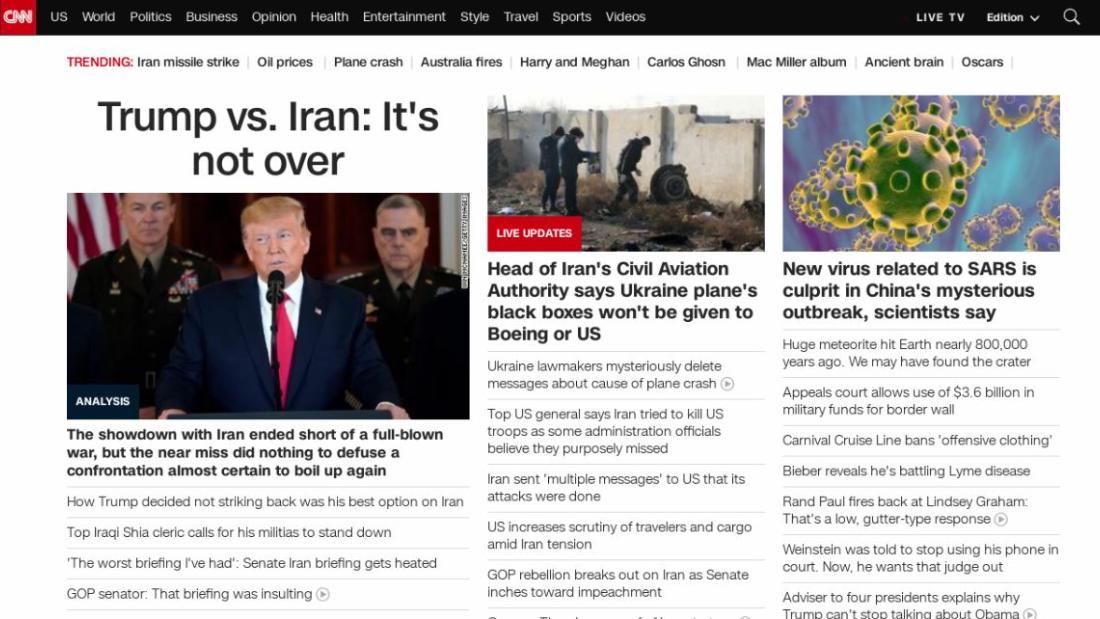The news website in the image is CNN. The top left corner features the "CNN" logo, which is written in white against a red background. Adjacent to the logo, on the right side, there are various header tabs with a black background and white text. These tabs, from left to right, are labeled: US, Wealth, Politics, Business, Opinion, Health, Entertainment, Style, Travel, Sports, and Videos. 

In the top right corner, there are additional options available, including "Live TV," "Edition," and a search button. Below these options, the section titled "Trending" is highlighted in red, while the trending topics listed beneath it are in black. These trending topics include: Iran missile strike, oil prices, plane crash, Australia fires, Harry and Meghan, Kellogg's cousin, Macmillan album, ancient Brian, and Oscars.

To the left side of the image, there is an article headline "Trump vs Iran is not over," accompanied by a picture of Donald Trump in a black suit, white shirt, and red tie. The subtext describes the situation between the US and Iran: "The short term with Iran ended short of a full-blown war but the near miss did nothing to defuse a confrontation almost certain to boil up again." Additionally, links to other related articles include: "How Trump decided no striking back was his best option on Iran," "Top Iraqi Shia leader calls for his militias to stand down," and "'The worst briefing I've heard': Senate Iran briefing gets heated, GOP senator says," with further descriptions about the briefing being insulting.

On the right side, another headline reads, "Head of Iran civil aviation authority says Ukraine planes black boxes won't be given to Boeing or US," followed by a subheading, "Ukraine lawmakers mysteriously delete messages about cause of plane crash." Additional headlines include: "Top US general says Iran tried to kill US troops, some administration officials believe they purposely missed," "Iran sent multiple messages to the US that its attacks were done," and "US increases scrutiny of travelers and cargo amid Iran tensions." 

There is also a headline about a GOP rebellion, "GOP rebellion breaks out on Iran and Senate turns to impeachment.” Below this, on the right, there's a headline about a virus: "New virus related to SARS is culprit in China outbreak, scientists say," accompanied by an image of a green virus. Subsequent news snippets include: "Huge meteorite hit near 800,000 years ago, we may have found the crater," "Appeals court allows use of $3.6 billion in military funds for border wall," "Carnival cruise line bans offensive clothing," "Pop star reveals he is battling Lyme disease," "Rand Paul fires back at Lindsey Graham: ‘There’s no cuter type response,’” "Winston told to stop using his phone in court, now he wants to charge out," and "Advisor to former president explains why Trump can't stop talking about Obama."